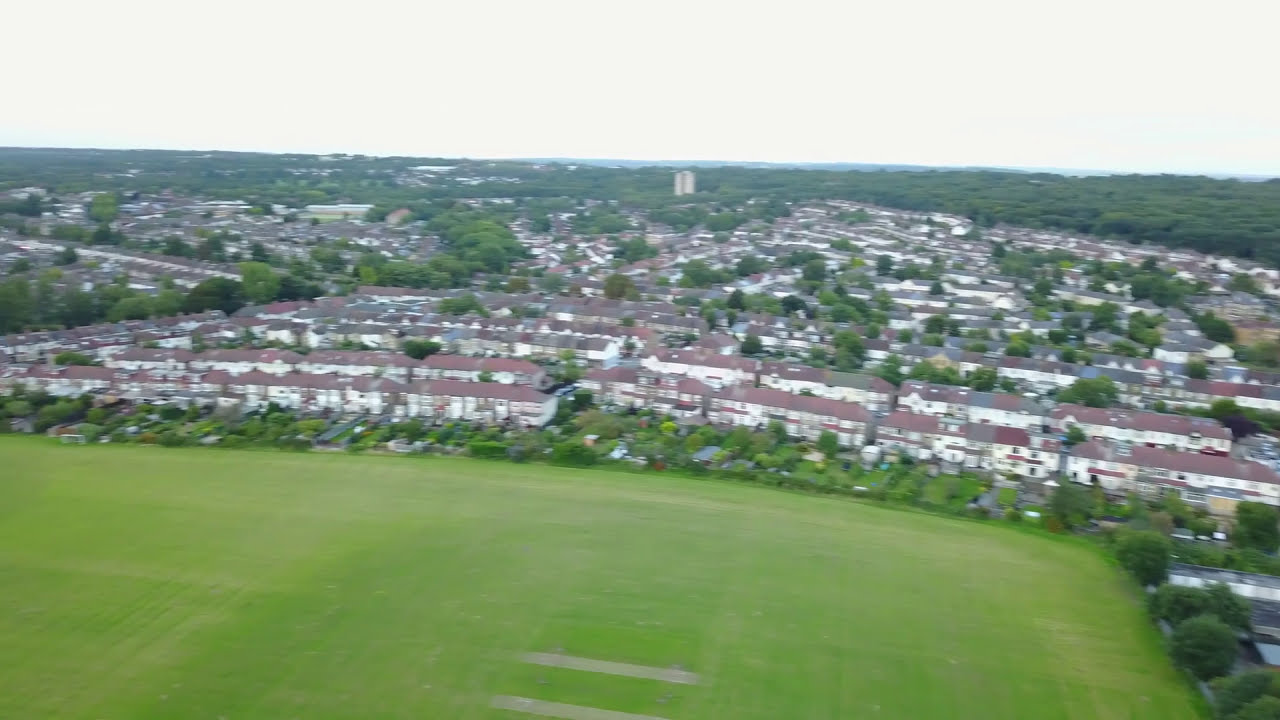Aerial view of a vast, meticulously manicured green field, situated in the bottom left corner of the image. The field is rectangular and could be a park or sports venue, with two faint gray tire marks near its center, suggesting some disturbance in the grass. Surrounding the field, a sprawling residential area is visible, featuring rows upon rows of identical white buildings with dark amber or red roofs, packed closely together. Interspersed between the buildings are occasional trees. To the right, a dense cluster of lush green trees is present, which could be a park or small forest, adding a touch of nature to the urban landscape. The horizon is marked by a hazy, almost white overcast sky, blending into the distance. The image is captured from a significant height, possibly by a drone, offering a broad perspective of the scene below.